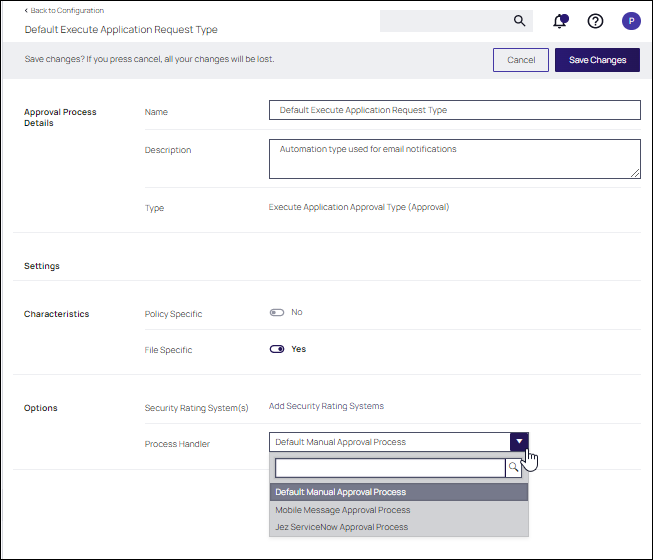The image portrays a user interface with a functional layout for configuring a BATU application. At the top, a search bar is positioned with the label "BATU Configuration" to its left. Below this section, there is an area labeled "Default Execute Application Request Type." Beneath this label, a gray box prominently displays the option to "Save Changes," with a cautionary note indicating that pressing "Cancel" will result in the loss of all changes. Both a "Cancel" button and a "Save Changes" button are situated in this section.

Further down the interface, on the left, there's a label reading "Approval Process Details." Adjacent to this on the right, the interface displays three columns. The top of the left column is labeled "Name," accompanied by an input box pre-filled with "Default Execute Application Request Type." Below this, the label "Description" is indicated, alongside another input box containing the text, "Automation type used for email notification."

The section continues with the label "Type," which specifies "Execute Application Approval Type (Approval)." Below this section, additional details are provided for configuration settings. The labels "Sentence Characteristics, Policy Specific" are presented with a toggle bar set to "No," and beneath this, "File Specific" is shown with its corresponding toggle bar set to "Yes."